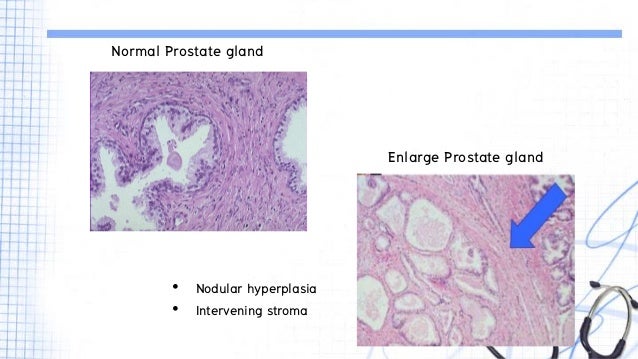The PowerPoint presentation slide provides a detailed examination of the male prostate gland using two microscopic images. The top-left section displays an image labeled "Normal Prostate Gland," exhibiting a whitish area encased by a purplish hue. Below this image, two bullet points read "Nodular Hyperplasia" and "Intervening Stroma," indicating specific characteristics or conditions associated with the normal prostate. On the bottom-right, another microscopic image is labeled "Enlarged Prostate Gland," featuring a blue arrow pointing from the top-right to the center of the image, emphasizing a particular area of interest. This image retains a similar color palette with slightly less purple. The slide is framed with blue-colored squares on the left and a solid blue line at the top. Additionally, the lower right corner of the presentation features the top part of a stethoscope and some blue squiggly lines, enhancing the medical context of the slide.